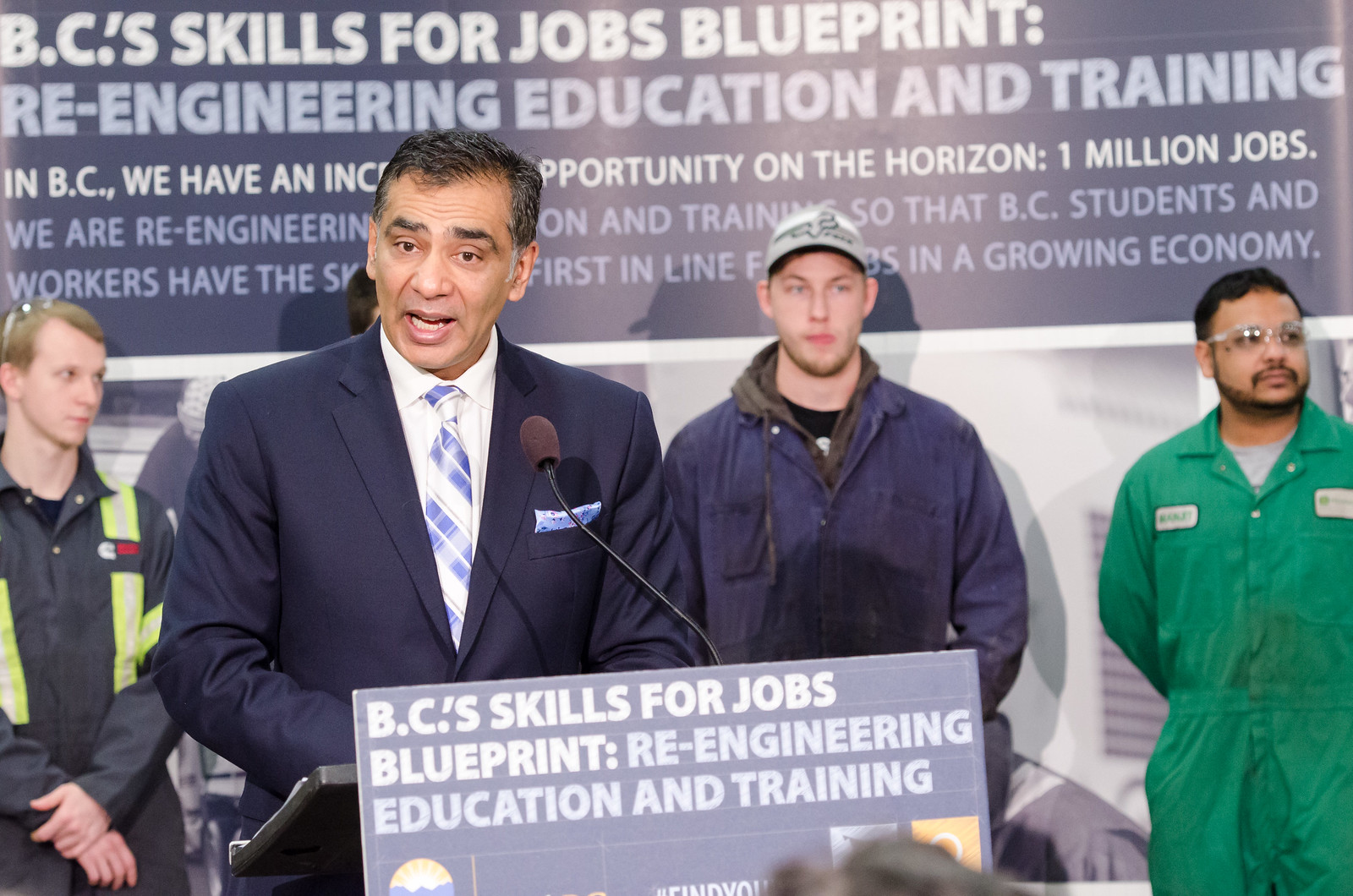The image depicts a middle-aged man with black hair graying at the temples, standing at a podium during what appears to be a news conference or public announcement. He is dressed in a navy blue suit, a white collared shirt, and a blue plaid tie. A neatly folded pocket square is visible in his breast pocket. The man is speaking into a microphone, possibly addressing an audience, and he appears to be in his late 40s to early 50s. His skin tone suggests he may have South Asian heritage.

The podium bears a sign that reads "BC Skills for Jobs Blueprint: Re-engineering Education and Training." Behind him, four individuals who look like trades workers stand in blue jumpsuits and high-visibility gear, with their hands either in front of them or behind their backs. One worker on the right is wearing clear glasses and a green jumpsuit. Their presence emphasizes the focus on skilled labor and training.

In the background, a prominent board also displays the slogan "BC Skills for Jobs Blueprint: Re-engineering Education and Training." The rest of the sign contains information about the initiative, mentioning the creation of one million jobs and the goal of positioning BC students and workers to be first in line for opportunities in a growing economy.